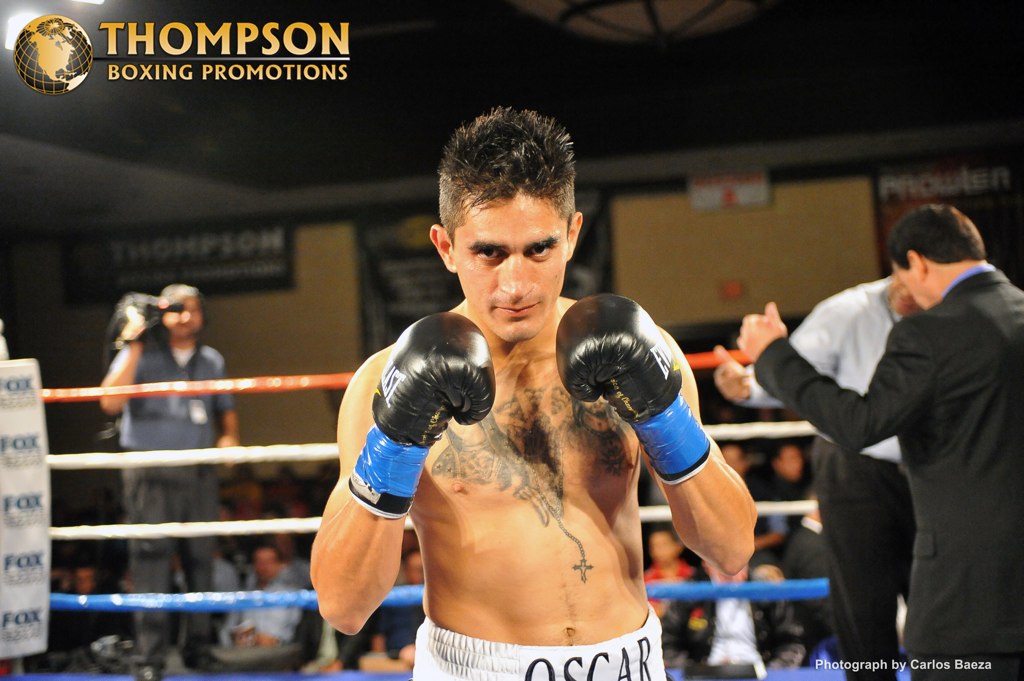This photograph captures a dynamic moment of a bare-chested, sweaty boxer named Oscar, standing ready in an indoor boxing ring. Sporting black boxing gloves with blue wrist tape, Oscar holds his fists up in a classic fighting stance, revealing a tattoo on his chest and a chain with a small cross above his navel. His white trunks prominently display his name "Oscar" in black letters on the front. The ring is defined by its four boundary ropes, colored orange, white, white, and blue from top to bottom, and an audience can be vaguely seen sitting blurred in the background. To Oscar's right in the ring are two more people, one of whom is a man in a dark suit talking to the referee, while outside the ring stands a cameraman capturing the action. In the top right corner of the image, a logo featuring a globe with gold latitude and longitude lines represents Thompson Boxing Promotions, with the text "Thompson Boxing Promotions" written in yellow nearby. At the bottom right corner, white text credits the photograph to Carlos Baeza.